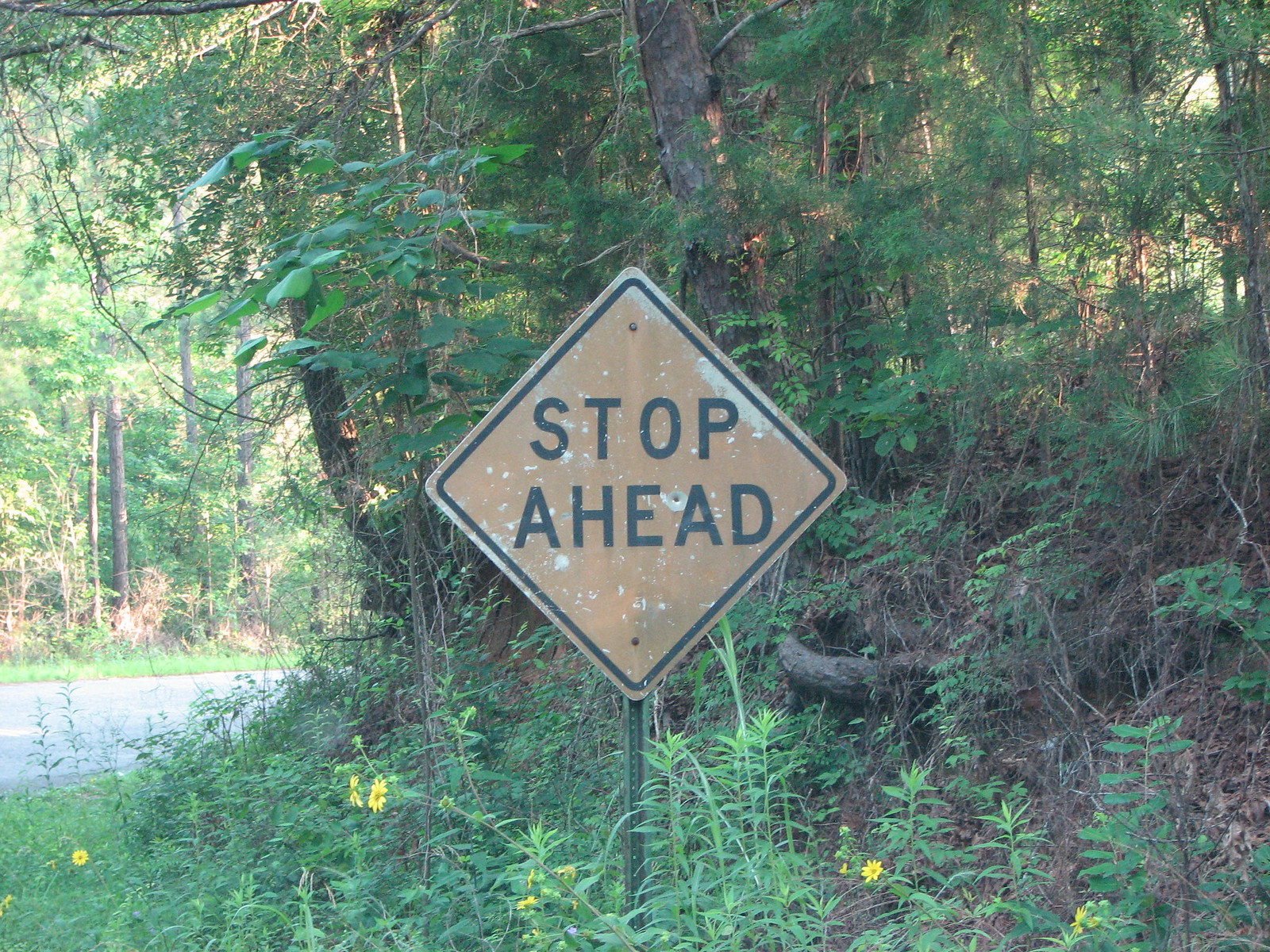A yellow, diamond-shaped "Stop Ahead" sign with black text and border is prominently displayed in a densely wooded area. The landscape features lush, verdant foliage, suggesting a location near a mountain or lake. The scene is bathed in sunlight, which filters through the trees in the background, casting dappled light onto the road and partially illuminating the area with greenery on either side. The foreground remains relatively shaded, contrasting with the brightly lit background, which emphasizes the tranquility and natural beauty of this serene, sunlit setting.